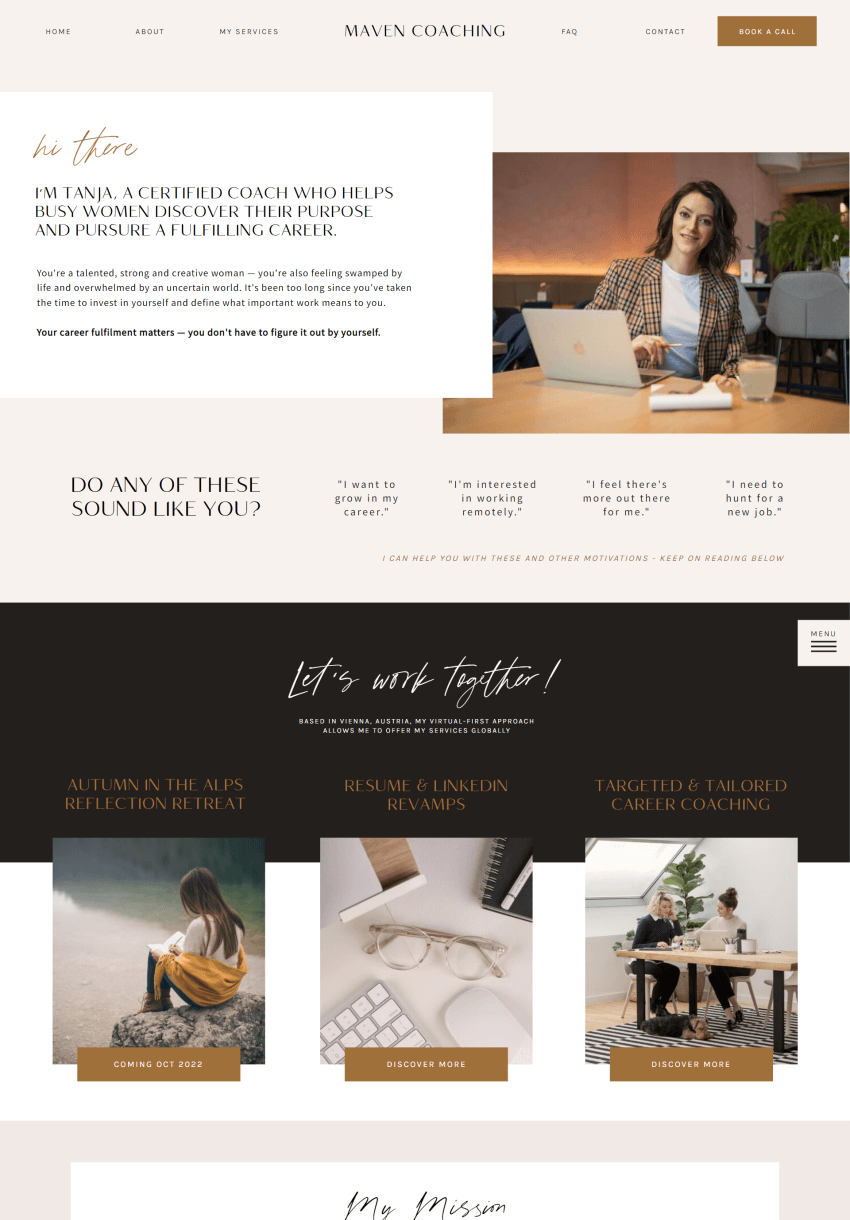In the image, the central focus is on a promotional banner for Maven Coaching. The header is beige with the Maven Coaching logo prominently displayed. A white square features an introduction from Tanja, a certified coach specializing in helping busy women uncover their true purpose and achieve fulfilling careers. 

The banner includes a photograph of a woman seated at a restaurant table, engaging with a laptop while enjoying a drink. On a beige rectangle within the image, the text poses a reflective question: "Do any of these sound like you?" followed by four quotes that capture common sentiments among Tanja's target audience.

Additionally, the banner contains a black rectangle with the motivating call to action: "Let's work together." Surrounding this section are three smaller images. The first depicts a woman sitting on a rock, absorbed in reading a book. The second image showcases a tidy workspace with glasses, a keyboard, a mouse, and a notepad with a white pencil laid out on a black surface. The third picture features two women engaged in conversation at a wooden table, emphasizing the collaborative and supportive nature of Tanja's coaching services.